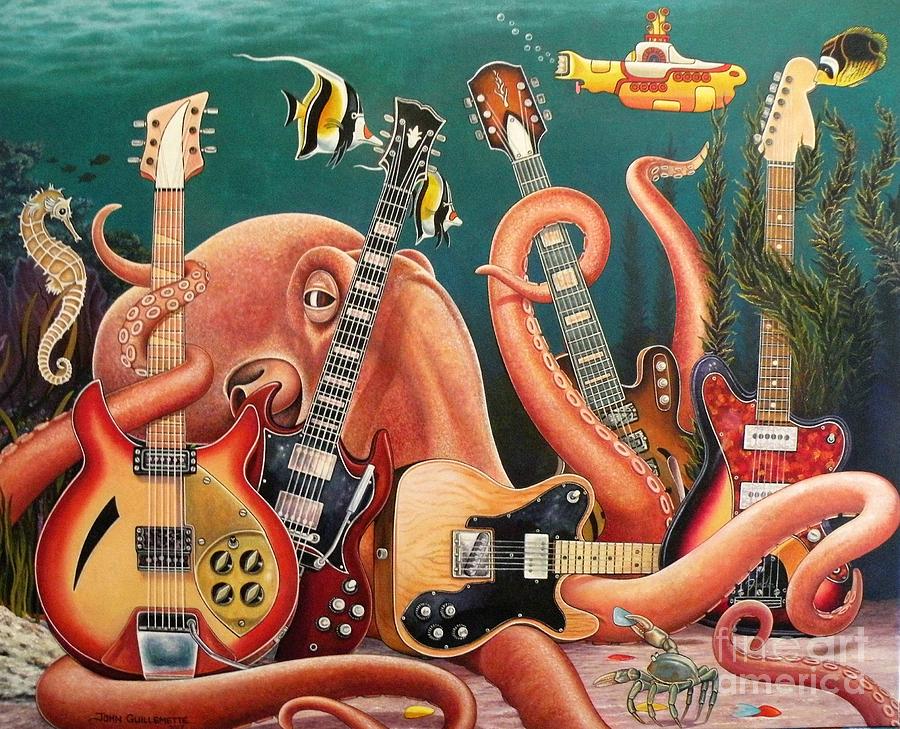This computer-generated illustration, inspired by the Beatles, features an underwater scene reminiscent of their "Yellow Submarine" film. Dominating the scene is a large octopus sitting on the ocean floor, with its tentacles wrapped around and playing five electric guitars. Above, the iconic Yellow Submarine is visible, adding a whimsical touch. Surrounding the octopus are various sea creatures: a crab holding a guitar pick, a curious seahorse gazing at the octopus, and several vibrant, yellow and black striped fish flitting around the scene. This artwork likely references the Beatles' song "Octopus's Garden," creating a vivid and playful aquatic world.